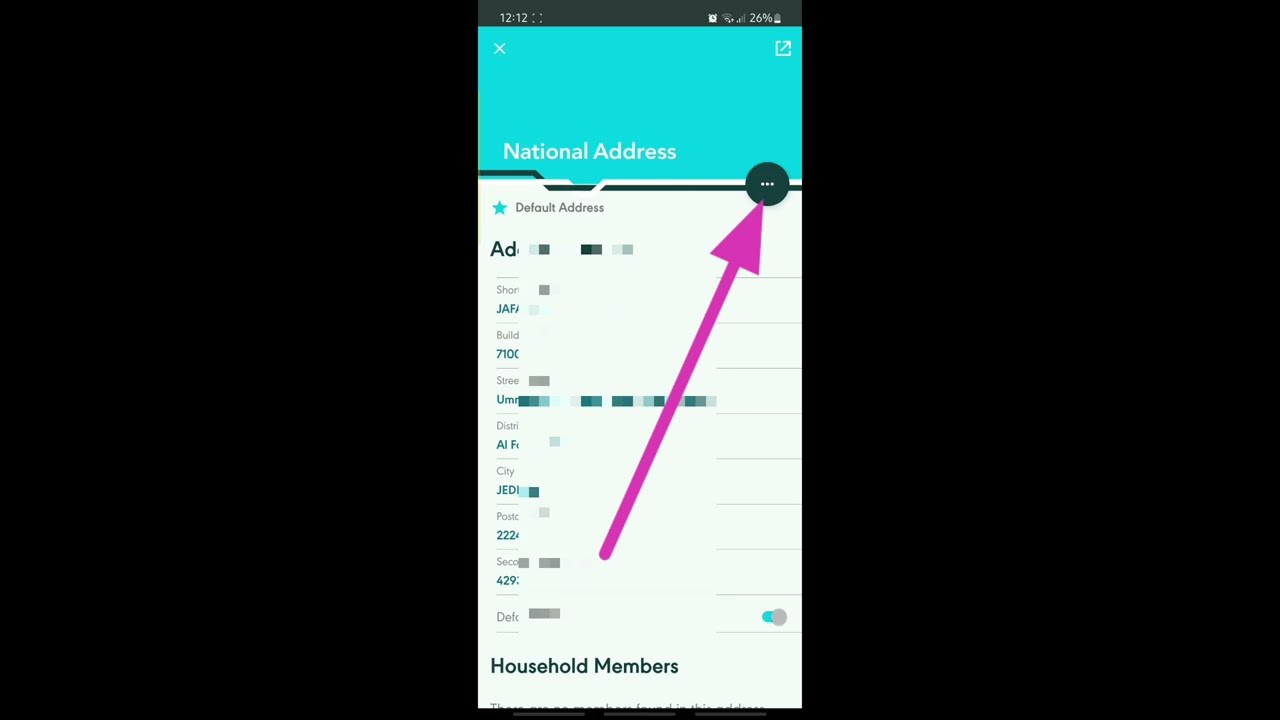This image is a mobile screenshot showcasing an app interface, framed in portrait orientation with black rectangles on the sides. The top bar reveals typical smartphone indicators: the time in the upper left, and icons such as the battery percentage and a clock in the upper right, confirming the mobile capture.

Dominating the top of the app interface is a blue header with "National Address" written in white text. Below this, a long white rectangle is prominently featured, labeled in black text at the top left corner as "Default Address," marked with a blue star.

A distinctive visual guide includes a large purple arrow pointing upwards towards a black circle with three white dots in the upper right corner, likely indicating a menu or settings option in the app.

Towards the bottom of the screenshot, black text reads "Household Members" near the left side. The address information in the app is blurred out, hinting at sensitive or private data while still maintaining the structural elements of an address book.

Overall, this detailed image seems to function as an instructional guide on how to navigate the app, marked by the arrow directing user interaction.